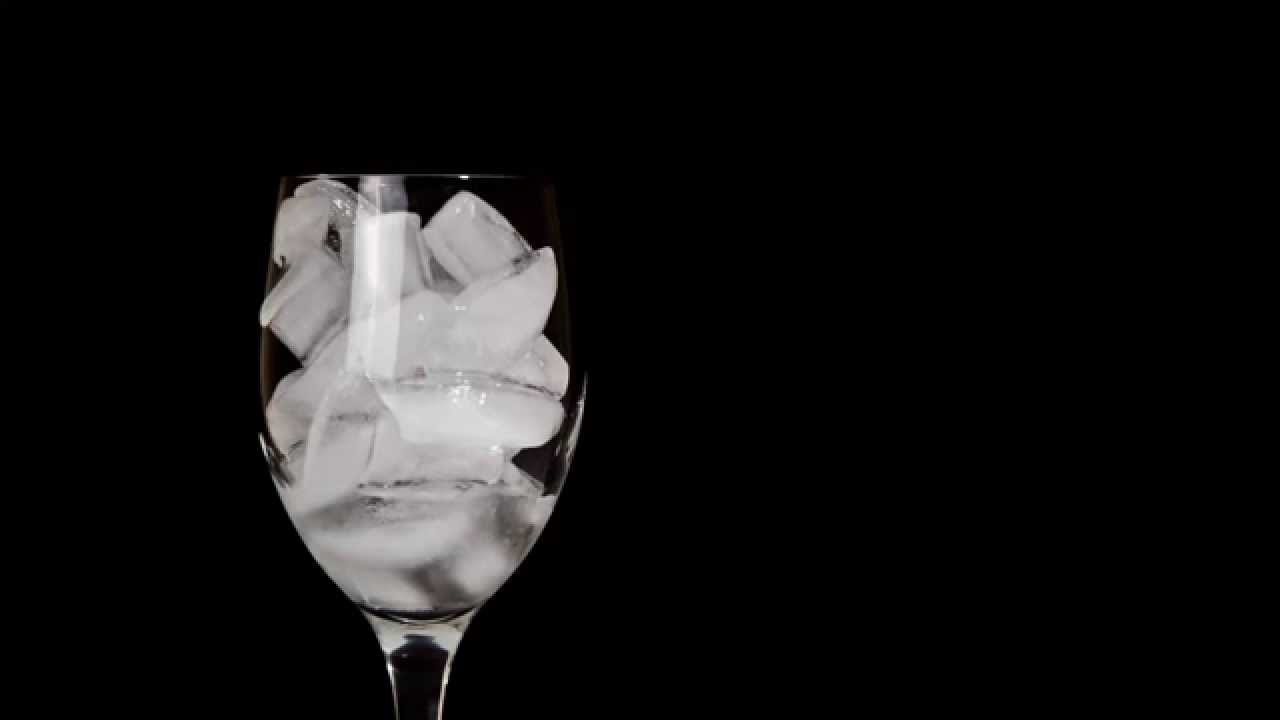In this image, set against a black background, there is a clear wine glass positioned toward the middle left. The glass, which is only partially visible, focuses on the upper part with a small portion of the stem shown. Inside the wine glass, it is filled to the top with elongated, white rectangular ice cubes. The ice appears to be melting, as evidenced by the accumulation of clear water at the bottom, filling about a fourth of the glass. A slight reflection of light highlights the well-lit glass, emphasizing the clarity of the wine glass and the melting ice within.